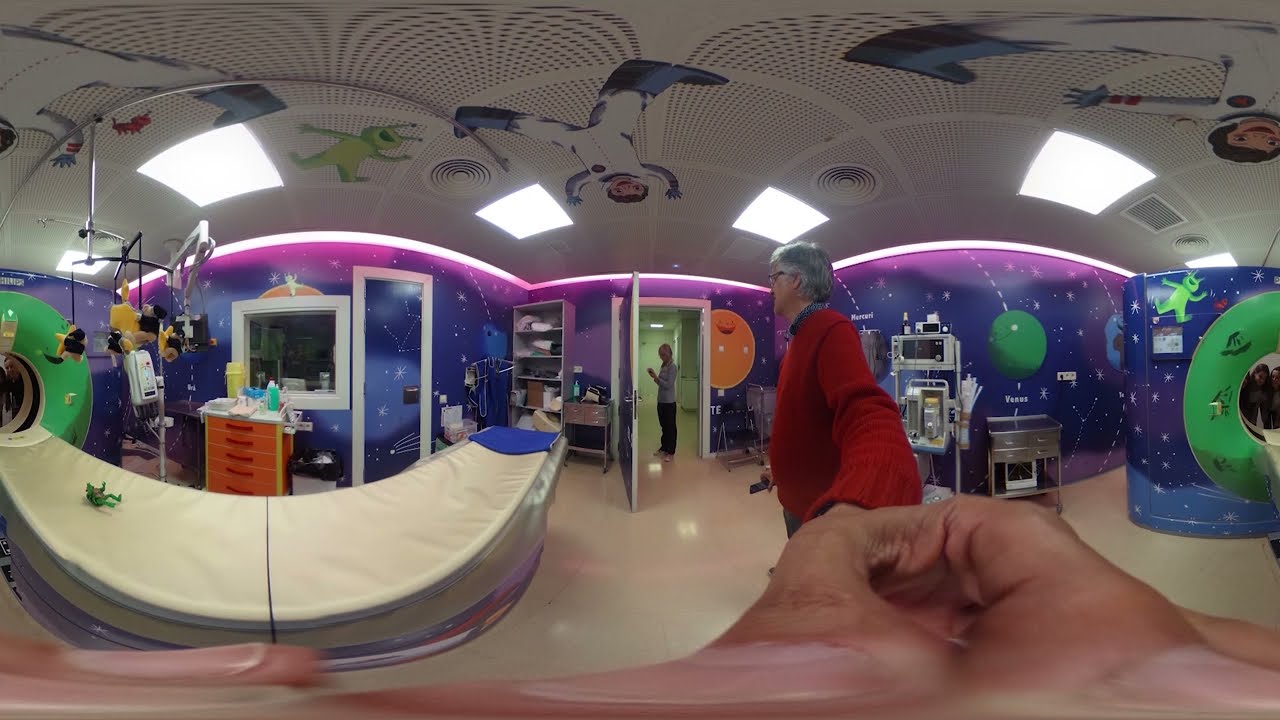The image depicts the interior of a children's hospital room, specifically designed to be inviting and comforting for young patients. The room is divided into separate, partitioned areas, each adorned with a vibrant space scene on the walls. The backdrop features a gradient from dark blue at the bottom to a purple ombre at the top, filled with illustrations of planets, stars, and green Martian monsters. The ceiling continues the theme, showcasing playful illustrations of aliens, frogs, and children in astronaut suits, all rendered in bright colors. Magenta fluorescent lighting further enhances the whimsical, celestial ambiance. In the foreground, a pair of cupped hands, slightly blurred, is directed towards a person standing near the front desk. This individual, identifiable by a red sweater, glasses, and short silvery-gray hair, is either an employee or a visitor, adding a human element to the scene. This setting might also feature an MRI machine, making it a multifunctional space within the hospital.